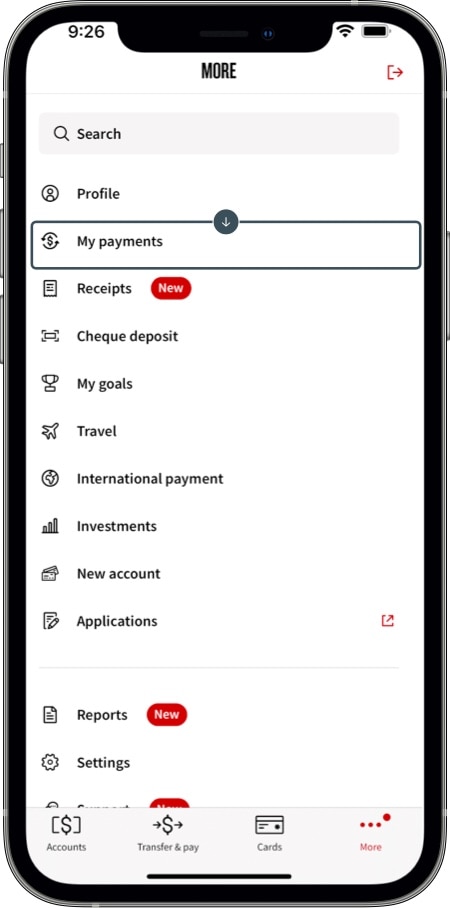This detailed image depicts a cell phone screen showcasing various app functionalities. At the top of the screen, the status bar displays the time as 9:26, a full cell signal icon, and a battery icon. Centered prominently is the text "More." Adjacent to this is a half-square icon with an outward-facing arrow, indicating an additional option.

Beneath this is a search bar, ready for text input, followed by a series of categorized navigation options. These options are displayed alongside illustrative icons: "Profile," "My Payments," "Receipts," "Check Deposit," "My Goals," "Travel," "International Payment," "Investments," "New Account," and "Applications." Each option is accompanied by a relevant image, such as a trophy for "My Goals" and an airplane for "Travel." Particularly notable is the red oval with white text reading "New" next to "Receipts." The "My Payments" category is prominently highlighted by a large square box, indicating it is currently selected. Similarly, the "Applications" option features the distinctive half-square icon with a red arrow, signifying an expandable element.

A separating line divides these sections from additional options below, which include "Reports" (also marked with the "New" indicator) and "Settings." At the very bottom of this screen, a gray pop-up-like section features further navigation buttons labeled "Accounts," "Transfer and Pay," "Cards," and a red button labeled "More."

The meticulous layout and intuitive icons make it easy to navigate through the functionalities depicted on the phone screen, ensuring an organized and user-friendly interface.